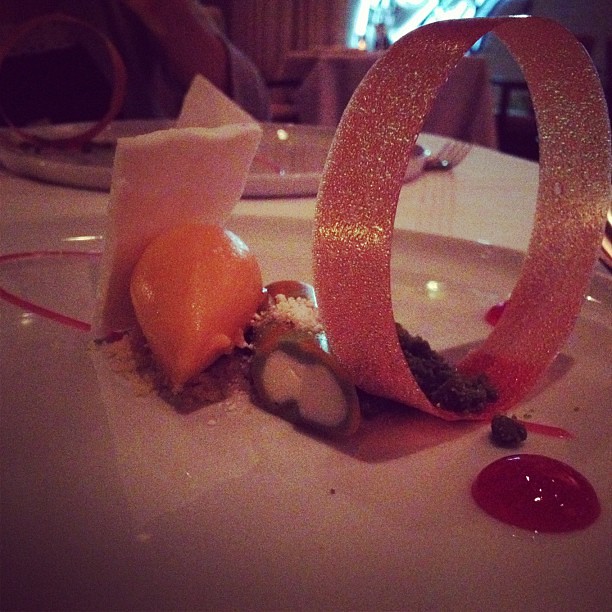In this low-light photograph taken at a high-end, expensive restaurant, the focal point is an intricately arranged dessert positioned at the center of a pristine white plate. The standout feature is a tall, shiny ring made from caramelized sugar, standing upright on the right side of the plate. Within and atop this ring is a brown, possibly nutty, substance that could be crushed pistachios. Centered on the plate is a rounded cylinder, green and orange, with a white interior, possibly a marzipan-filled candy.

Adjacent to this is a vibrant, orange, teardrop-shaped object, likely a fruit purée or gel, and leaning against it is a sharply angled, white rectangular piece resembling a small book. Scattered around the arrangement are smears of vivid red sauce, delicate black and white crumbs, and what looks like a glossy red mass. 

The background reveals the elegant setting of the restaurant, adorned with tan curtains and a person steps through an illuminated area suggestive of a window or doorway. White tablecloths, dark wooden chairs, and another diner with a similar dessert enhance the sophisticated ambience. This diner, wearing a gray and black outfit, is positioned closer to the left, with neatly stacked plates and silver forks adding to the scene's refined details.